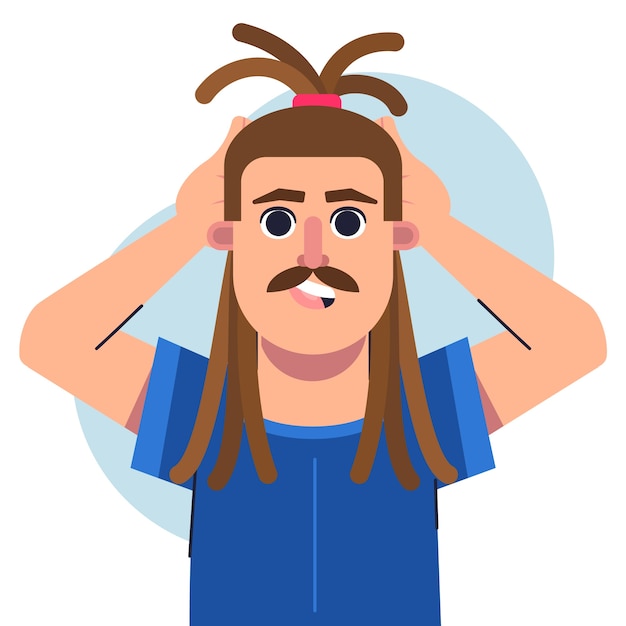The image depicts a detailed cartoon illustration of a light-skinned man with long brown hair tied into a ponytail that rests on his shoulders. He has a thin, brown mustache, bushy eyebrows, and large black eyes. His mouth is open, revealing white teeth, and his expression is slightly crooked. He is wearing a blue shirt with darker blue in the body, while the sleeves, neckline, and center are a lighter blue. His hands are positioned behind his head, as if in the midst of tying his hair up. The man stands against a background consisting of a large blue bubble, with the rest of the backdrop being white. The image gives off a playful and artistic vibe, reminiscent of digital artwork created using a computer drawing program or a tablet.